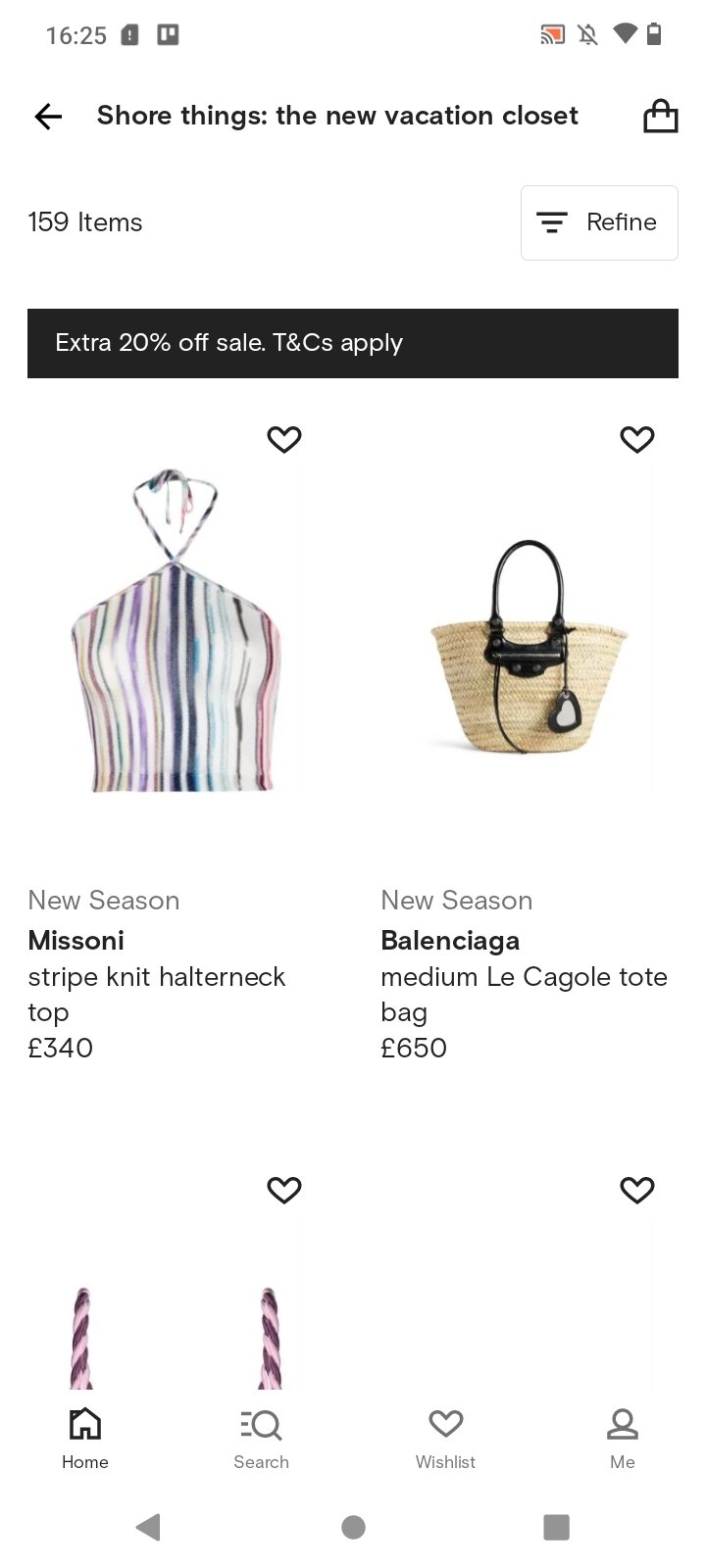Here is a detailed and cleaned-up caption for the given image description:

---

A screenshot captured from a tablet or smartphone webpage is depicted, identifiable by the notification bar at the top. The time displayed is 16:25 in military format. The notification bar includes icons for an SD card, a screenshot, a cast feature (illustrated by a black square with orange interior and wireless rays), a muted notification bell, a strong Wi-Fi signal, and a battery level slightly over half full. 

Below the notification bar, on a white background, a black left arrow is visible. Bold black text reads "Sure things... The new vacation closet." To the right, an icon of a bag and a shopping cart symbol can be seen. Below this header, the text "159 items" is displayed. On the right side, there's a white button with black text, featuring three cascading lines and labeled "Refine," indicating filter options.

Further down, a black rectangle with white text reads "Extra 20% off sale. T&C's apply." Underneath this promotion, product images are displayed. The first image on the left resembles a bag or top, striped with yellow, purple, blue, green, and red. The gray text below it states "New Season," followed by "Missoni" in bold black text. The product description "Striped knit halter neck top" is listed with a price of 340 euros or pounds.

Next is an image of a tan bag with a black handle and a heart-shaped tag, black on the exterior and white on the interior. It is labeled "New Season," with "Balenciaga" in bold black text. The description "Medium Le Cagole Tote Bag" follows, priced at 650 pounds. Lastly, there's a partial view of a tank top or shirt with bands of maroon and pink, cropped off at the shoulder. 

---